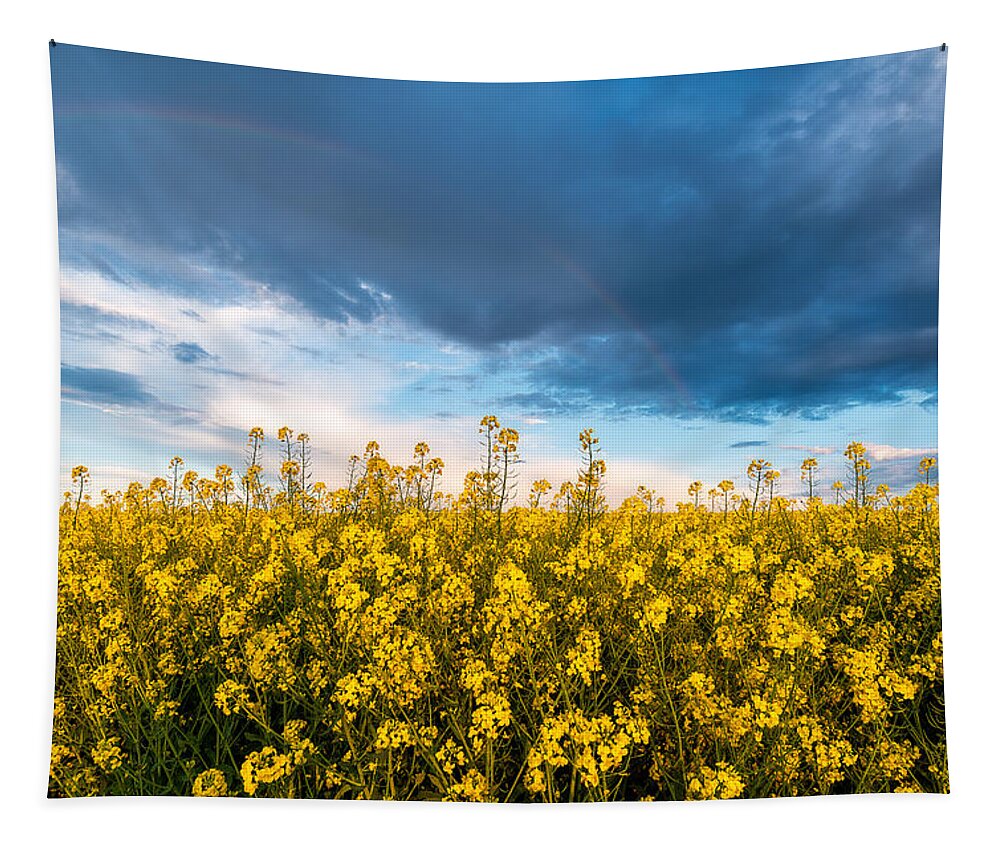A breathtaking landscape showcases an extensive field of vibrant yellow flowers, some of which appear to be slightly dried out. The flowers, standing tall, create a sea of yellow that blankets the bottom portion of the image. Towering above this field, the sky is painted with a mix of stormy blue clouds and fluffy white clouds, contrasting beautifully with the golden hues of the flowers. The blue clouds, heavy with moisture, hint at an impending storm, while the white clouds add a sense of lush tranquility. The scene exudes a raw, natural beauty, capturing the serene yet dynamic interaction between the land and sky.